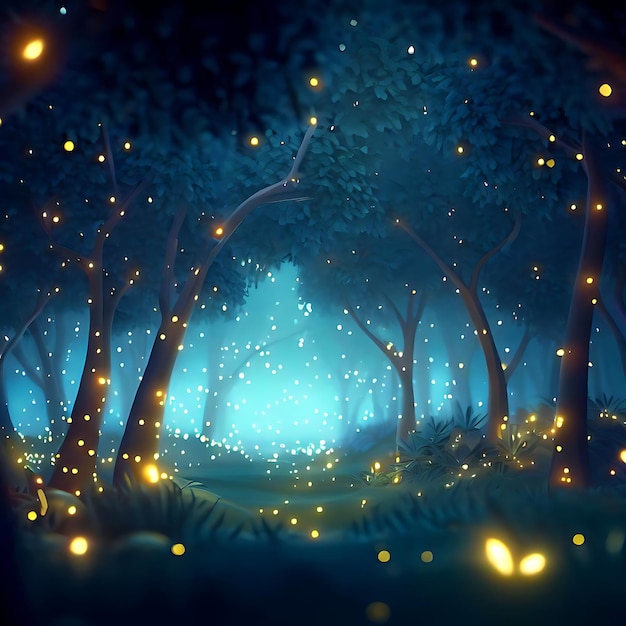The image is an artwork depicting a serene nighttime forest filled with the enchanting glow of countless fireflies. The scene showcases trees with bare bark halfway up, crowned by green leaves at the top. The forest floor is covered in slightly tall grass, which appears lush and green despite the night setting. The artwork employs hues of light blue and darker bluish green to create a mystical atmosphere, punctuated by very dark tones around the edges of the image. The trees appear somewhat blue due to the interplay of dim night light and the glow of the fireflies, which are represented as perfect small, circular dots in a yellowish color, numbering potentially in the hundreds. In the back part of the image, a white bluish light illuminates the scene but does not overshadow the twinkling fireflies. Overall, this detailed and color-rich artwork captures the enchanting beauty of a firefly-lit forest night, presenting a magical and serene outdoor setting.